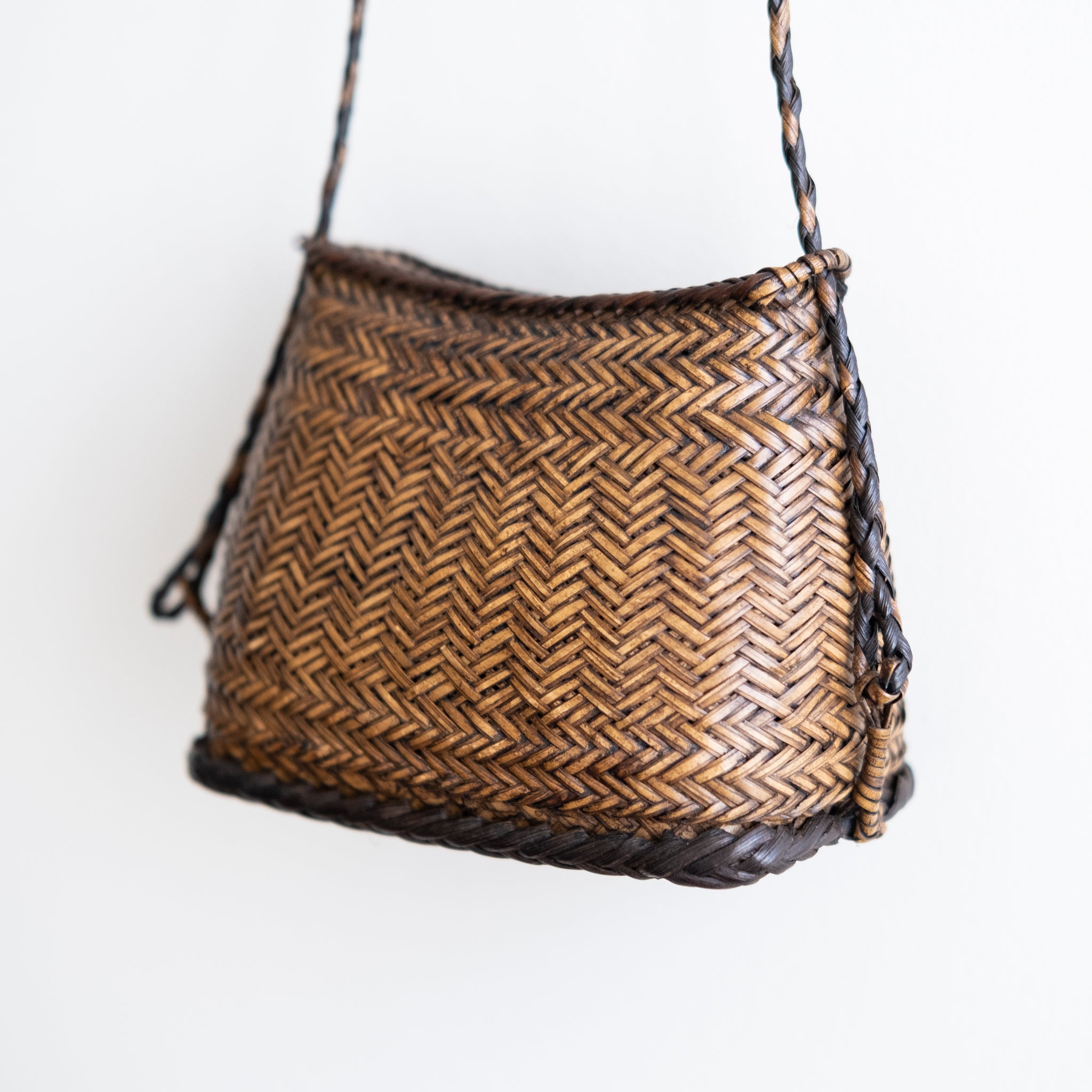This image showcases a vertically rectangular, intricately woven basket with an emphasis on its detailed craftsmanship. Set against a pale bluish-gray indoor background, the close-up reveals a basket that could easily be mistaken for a woven purse due to its delicate design. The basket features a base accentuated with dark black, thickly woven material, and is adorned with alternating light brown and black woven strands. Starting from the bottom, above the black base, two horizontal woven lines encircle the basket, followed by a series of vertical woven patterns resembling beads. Higher up, three additional horizontal woven lines round the top section. The basket's structure widens towards the bottom, enhancing its robust feel, while the top narrows slightly, creating a conical shape. Both sides of the basket sport long woven straps, composed of interlaced light brown and black wicker, each anchored by metal loops. These straps, although disappearing out of the frame, suggest a possible use as a hanging or carrying feature. The varying weaving patterns, from zigzags on the upper body to chevrons pointing downward at the center, highlight the basket's meticulous and resilient construction, hinting at its capacity to bear significant weight.